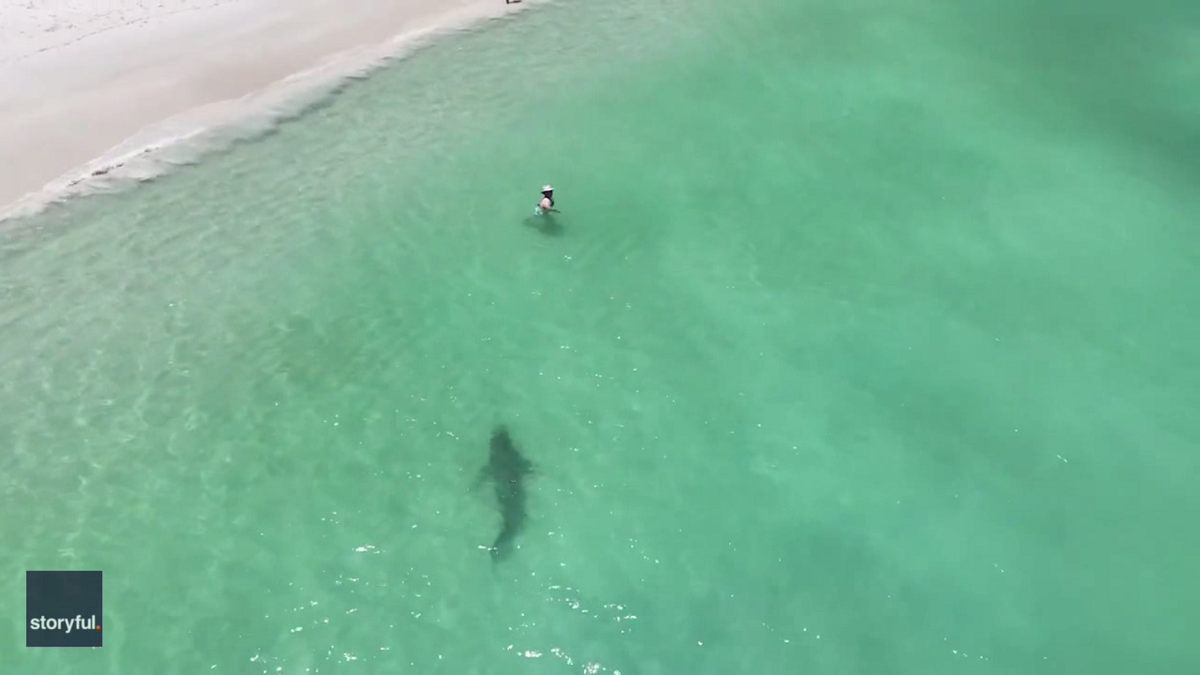In this horizontal image by Storyful, we see a detailed aerial view of a tropical shoreline. The clear, green waters gradually lighten near the white sandy beach, which occupies the upper left-hand corner. There's a single individual in the water, who appears to be either swimming or standing in the shallow ocean. Further below this person, towards the lower center of the image, the dark shadow of a large shark looms, seemingly swimming towards the unaware swimmer. The water in the upper right-hand corner is a darker green, while some gray patches are visible near the shoreline. In the lower left-hand corner, there is a black square with the text "Storyful" written in white.